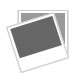The image is a horizontally oriented, rectangular illustration resembling a business card and serves as a poster or advertisement for an anime. In the upper center, "SHIRO FUBUKI" is prominently displayed in all caps white text, accompanied by four Japanese characters beneath it. The upper right corner features the letters "FW" in red alongside four yellow stars and a copyright symbol followed by some text that appears blurry. 

On the left side, there’s a running anime-style character with short, spiky purple hair and large green eyes. She has a heart-shaped face with a tiny mouth and nose. The character is dressed like a soccer player, wearing a white long-sleeved shirt with a gray collar and Japanese characters across it, paired with gray shorts that have white stripes along the sides. She sports a green armband around her upper left arm. Behind her, there is a jagged blue lightning strike outlined in white. The background is a mix of black diagonal lines with bluish-gray tones.